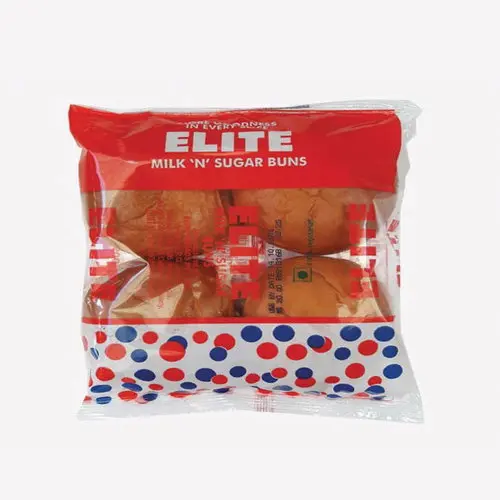The image showcases a square package of Elite Milk and Sugar Buns against a pure white background with no border. The packaging consists of four brown buns with creases on their tops, clearly visible through a central clear plastic section. The top portion of the package is red with white lettering that reads "Elite Milk and Sugar Buns." The center section features red vertical text that says "Elite" and also includes some black writing that appears to be the date and expiration information. The bottom of the package is white adorned with red and blue polka dots. The entire package is sealed and prominently displayed in the middle of the image.